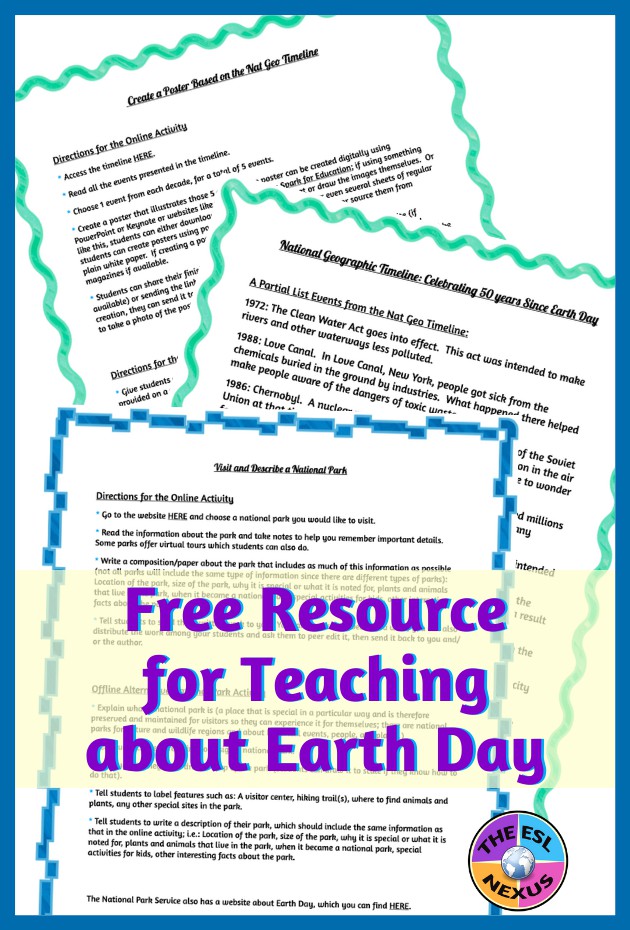Three overlapping pages are depicted in this image. The middle and back pages feature a green squiggly outline, while the top page is adorned with a blue checkered border. The image itself is framed with a solid blue trim. Across the top, a line resembling masking tape bears the words "Free resource for teaching about Earth Day" in striking purple text. In the bottom right corner, "The Thesal Nexus" is prominently displayed.